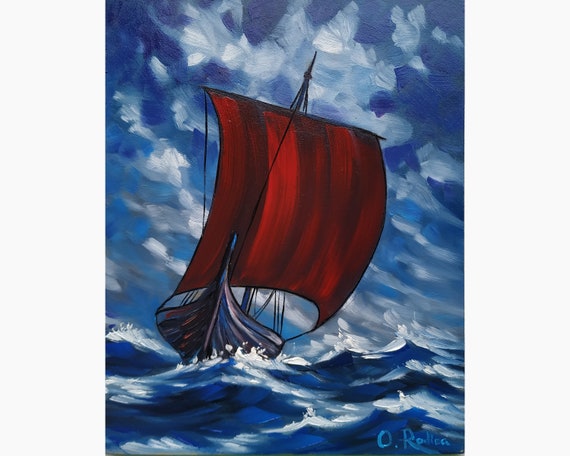This detailed painting, rendered in portrait orientation, depicts a Viking longship navigating through choppy, dark blue waters with visible white caps. The wooden vessel, light brown with dark blue and brown sections, occupies the left side of the image and is leaning to the right, pointing towards the viewer. A striking large red sail, unfurled and billowing convexly to the right, dominates the scene, with its mast extending above the sail. The sky is a gradient of medium to light blue, adorned with white cumulus clouds stretching diagonally from the top left to the bottom right. The painting's style is color oil, and it includes a signature in the bottom right corner, reading "O.R.O.L.L.E.A." in white. The scene is imbued with dynamic colors including ocean blue, sky blue, and various shades of white, capturing the essence of an ancient seafaring adventure. Text inscribed within the image reads, "Oh Rosa Rosa."